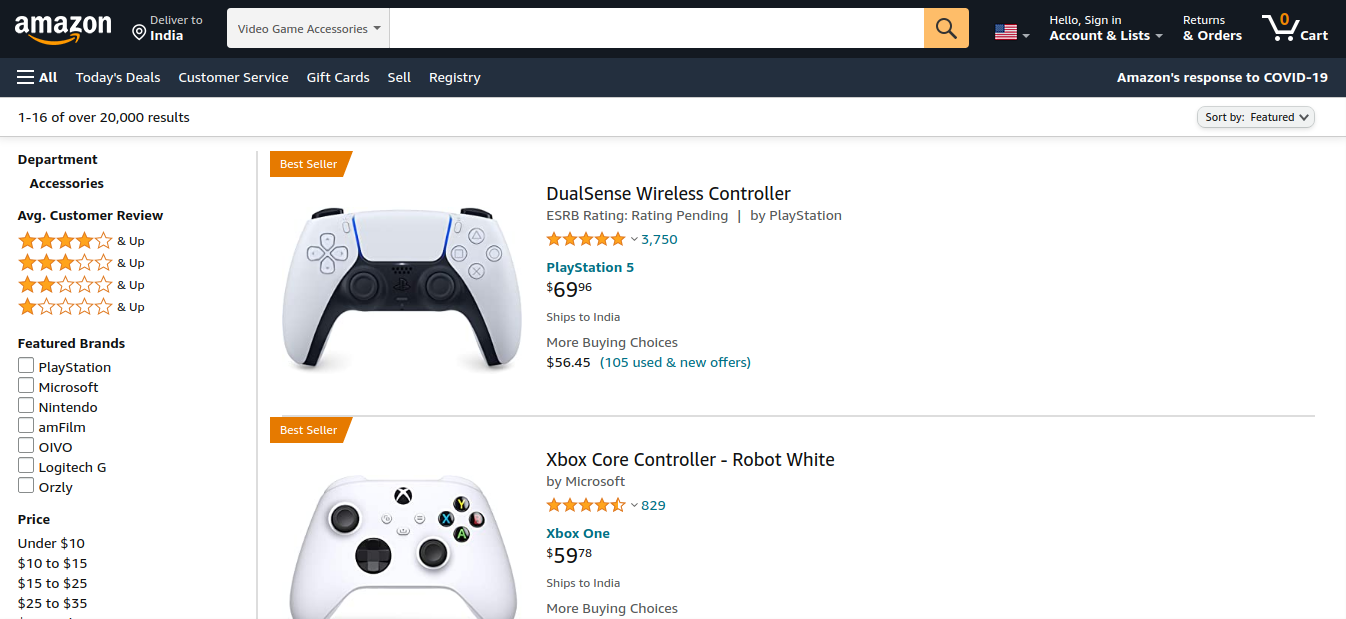In the provided screenshot, a user has captured a search result from Amazon, a prominent e-commerce platform. The search is filtered for video game accessories, specifically within the Indian region, as indicated by the "Delivered to India" label in the top left corner of the screen. The user is navigating through a subsection dedicated to this category, which includes items ranging from controllers to headphones, among other accessories associated with video gaming.

The image highlights two prominently featured products, each marked with Amazon's "Best Seller" badge. The first product is a PlayStation 5 DualSense wireless controller, a popular accessory for the latest generation of Sony's gaming console. Directly below it is an Xbox Core controller in 'robot white,' sold by Microsoft. Notably, the Xbox controller is priced at $59, which is $10 less than the DualSense controller, reflecting a slight price difference between the two leading gaming brands. This juxtaposition offers an interesting point of comparison for potential buyers.